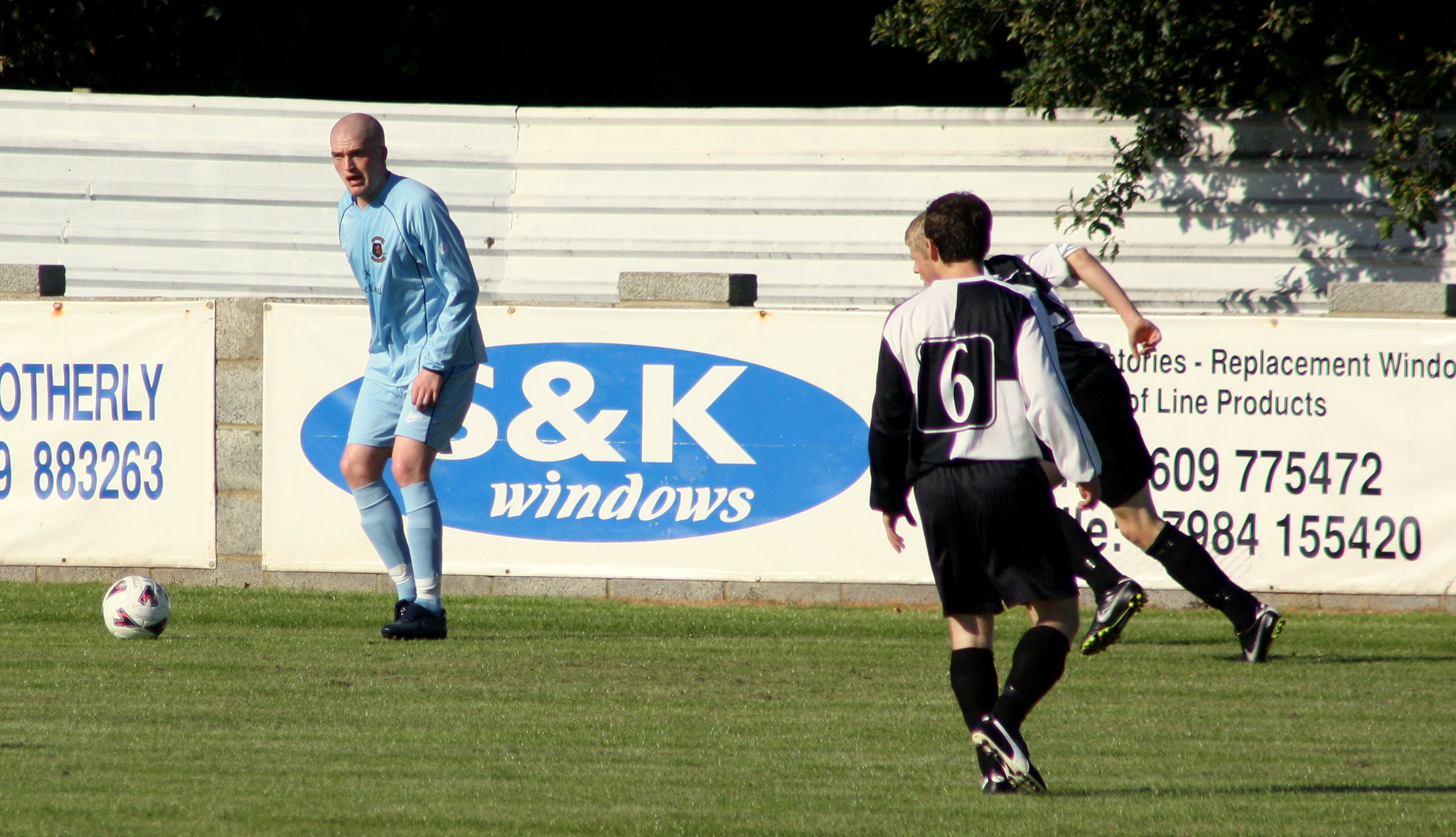In this vivid outdoor photograph taken during the daytime, we see three soccer players on a vibrant green grass field, indicative of a soccer pitch, with a background comprising a concrete block stone wall adorned with various advertisements. The wall displays a blue oval with the letters "S&K" and "Windows" beneath it, while another advertisement partially reveals words like "replacement," "window," "products," and a phone number, although some digits are obscured.

In the foreground, positioned closest to the viewer, a player with short dark hair stands with their back to us, adorned in a black and white checkered jersey featuring black shorts and black knee-high socks. Behind them, another player, whose blonde hair is slightly visible, appears mid-stride, also sporting black shorts and a black and white sleeve, indicative of similar team attire.

To the left of these players, a man, possibly part of the game or a coach, is dressed in a full light blue uniform, including a long-sleeve shirt, shorts, and knee-high socks. He is bald and seems poised to kick a soccer ball placed in front of him. Above the wall, a silver corrugated metal barrier extends horizontally, with a tree's foliage just overhanging it on the upper right section of the image. The upper left-hand corner features a darker background, contrasting with the silver barrier and vibrant green field below, visually anchoring the dynamic action of the soccer game.